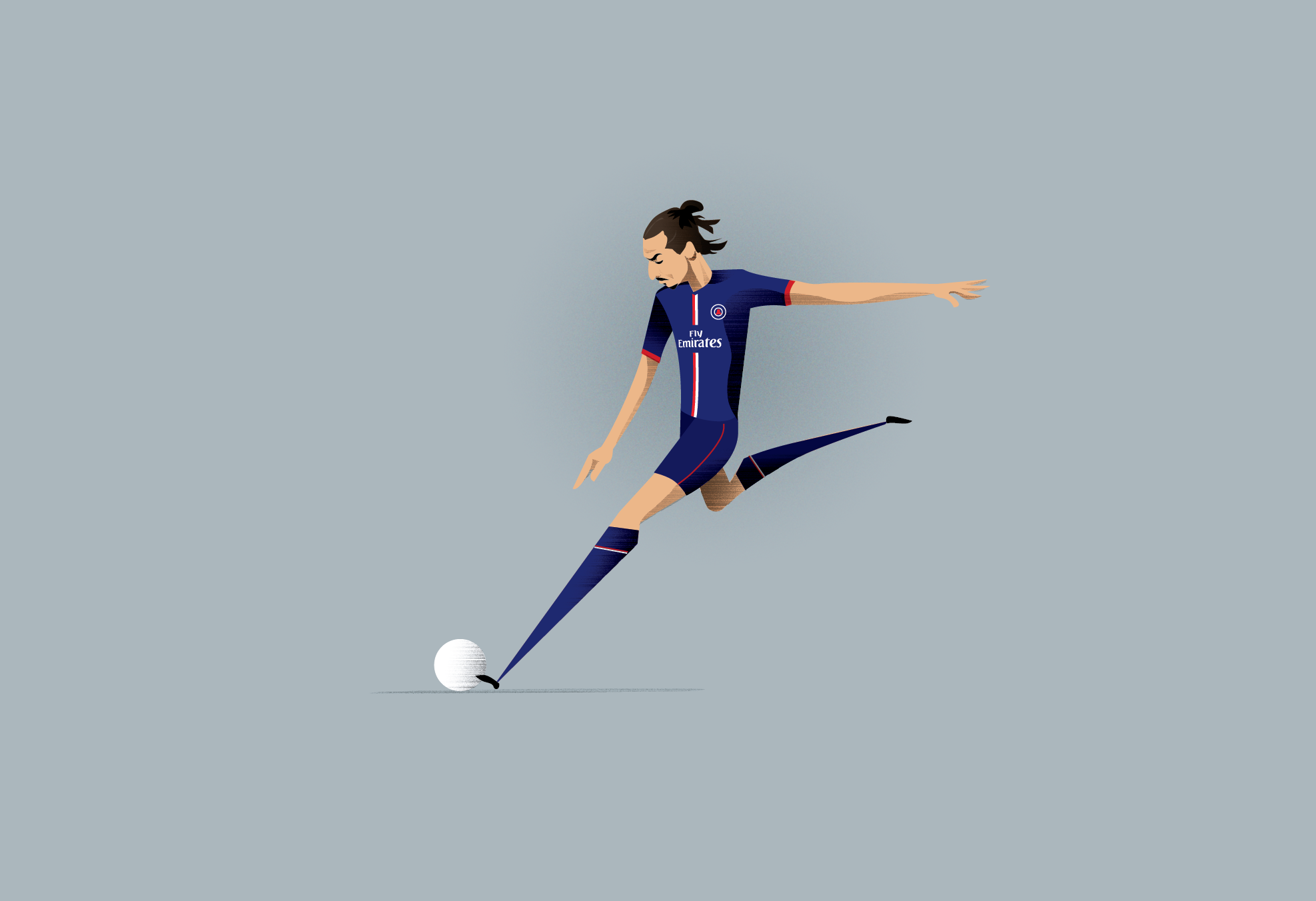The image is a digital illustration of a soccer player, set against a solid gray background. The character is depicted with exaggerated dimensions, featuring unusually long, thin legs, and disproportionately tiny feet, which adds a slightly eerie quality to the artwork. The soccer player is captured in mid-motion, running towards the left side of the frame with one leg bent backward and the other extended forward, kicking a ball.

The player is dressed in a detailed uniform, consisting of a blue top with black accents along the sides and a distinct vertical red and white stripe down the center. The sleeves reach halfway down his biceps and end in red cuffs. The jersey also has some white writing in the center, with the word "Emirates" discernible among the lettering. The top right of the jersey features a symbol resembling a bullseye, composed of concentric rings in white and blue, with a red dot in the middle.

He wears darker blue shorts, either shadowed or a darker shade, with a red stripe down the center, and long knee-high blue socks, which bear horizontal red and white stripes just below the knee. The player's facial features include a mustache, a concentrated expression, pronounced brows, and a man bun, enhancing the character's distinctive appearance.